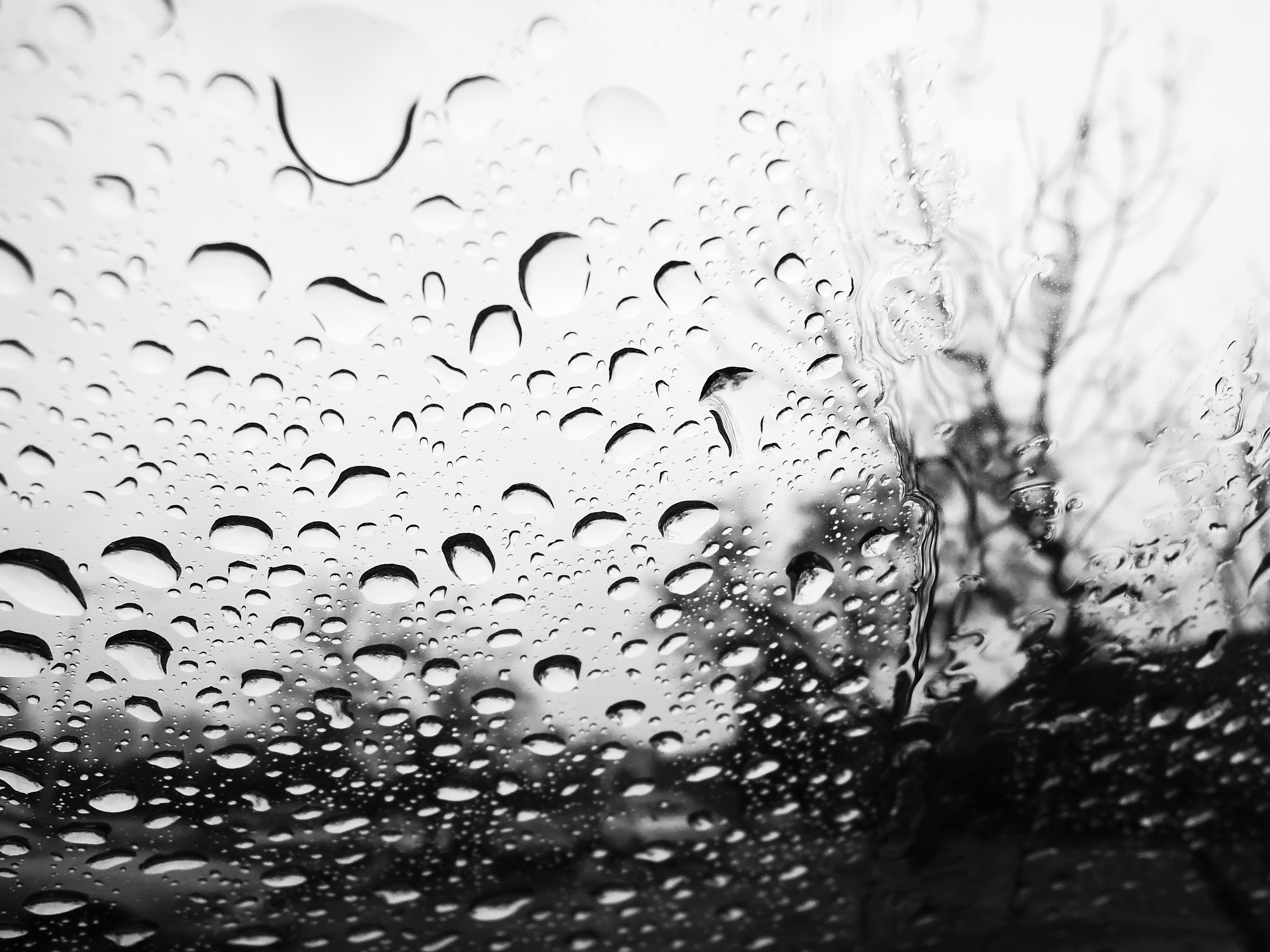This black and white image captures the view from inside a car, looking up through a slanted windshield covered in hundreds of water droplets, suspended after a recent rain. The droplets cling to the clear glass, with one area distinctly wiped clean, creating a streak that resembles a small river. This cleaned area might be the result of a windshield wiper, a hand swipe, or simply a natural run-off. The background outside the car is highly blurred, featuring the faint outline of leafless trees, suggesting an overcast day. The entire scene evokes a quiet, rainy atmosphere.